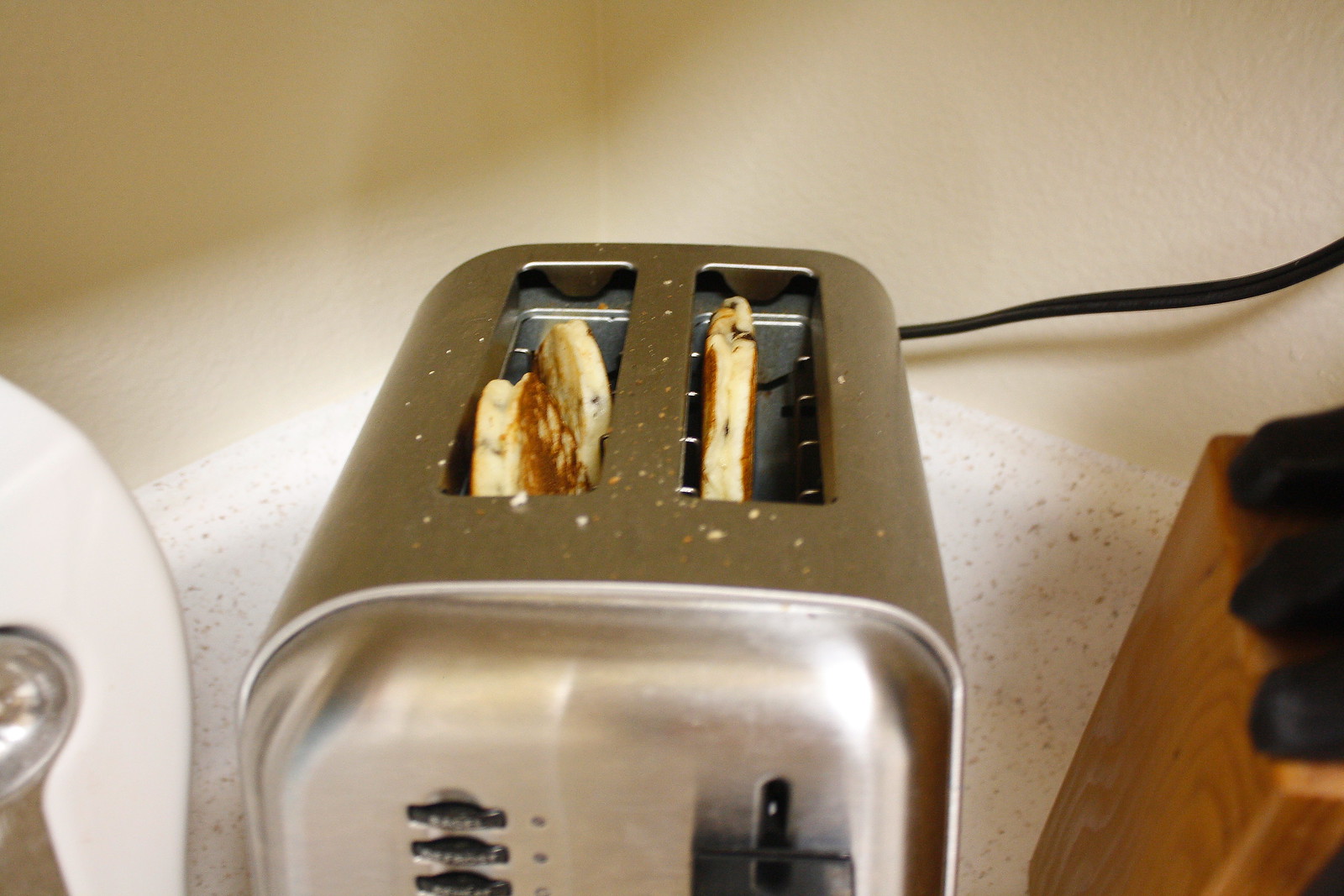The image captures a detailed kitchen scene centered around a silver, vintage-style toaster positioned on a speckled white countertop. In its two slots, there appear to be pancakes, accompanied by scattered crumbs on the surface around the slots, contributing to a slightly untidy look. The front of the toaster is adorned with multiple buttons labeled in white. Behind the toaster, the power cable extends off to the right side of the image. To the left of the toaster, a partially visible white appliance with a silver chrome section peeks into the frame, while to the right, a wooden knife holder with black-handled knives is clearly visible. The backdrop consists of a corner made by two mostly white walls, distinguished by black speckling near the bottom half, adding a subtle contrast to the scene.